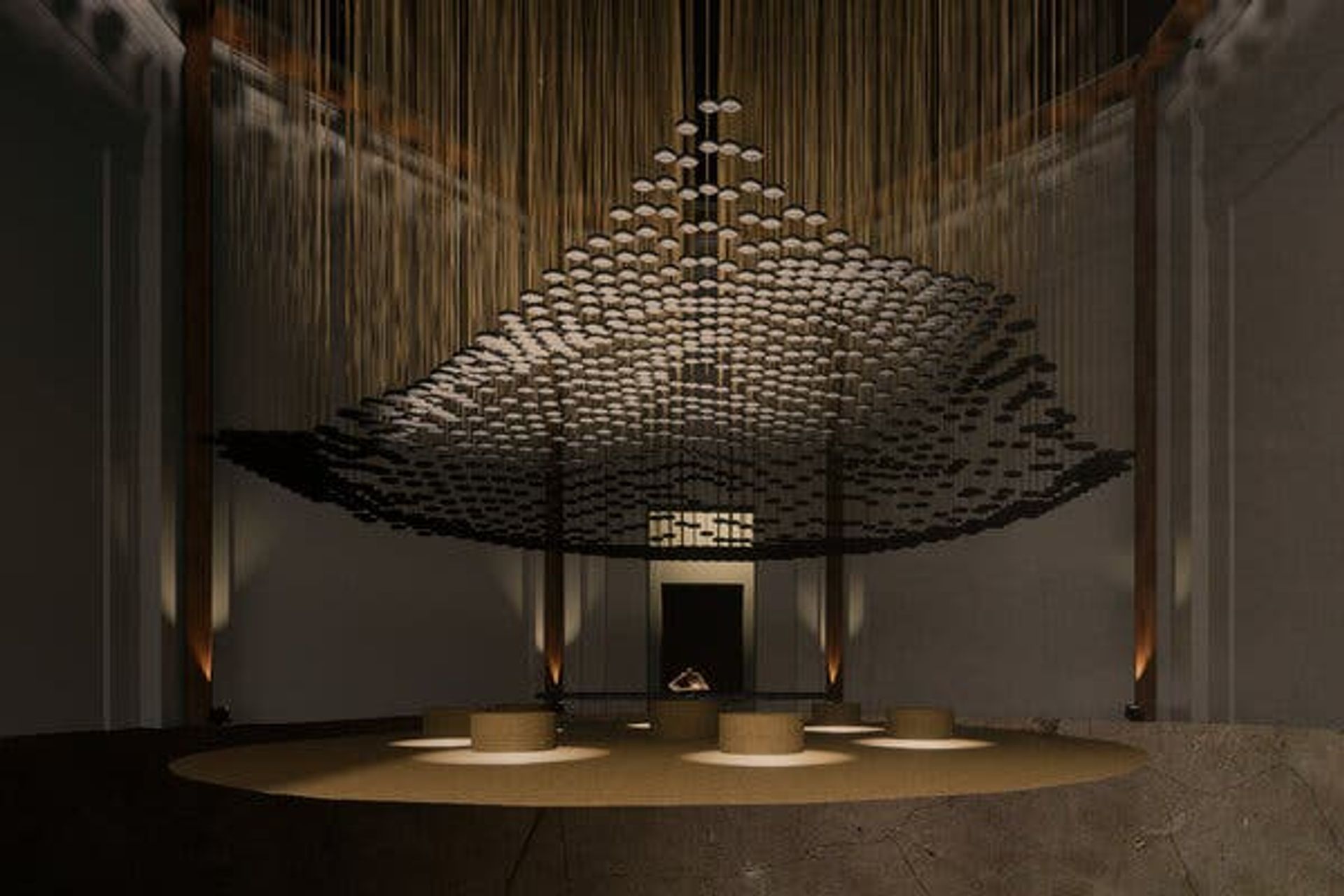A photograph of a dimly lit, spacious interior, possibly a modern art museum or stage, characterized by its high ceilings and minimalist design. The ground is dark and cracked, appearing to be cement or granite. Centrally positioned is a lighter beige area featuring four large, cylindrical, half-cylinder-like seats arranged in a circular pattern. Above these seats, a black canopy with numerous small, white sections dangles overhead, resembling hanging strings with attached circles, creating a mountain-like or triangular pattern in the sky. Ambient light from the ceiling illuminates this central arrangement. The background walls are gray, with faint, gold streaming lines descending from the ceiling. A notable feature in the back is a black doorway framed in silver metal, adding to the modern aesthetic. The overall color palette of the scene is dominated by shades of brown, gray, and white. The space is devoid of people and other objects, emphasizing the serene and contemplative atmosphere of the installation.